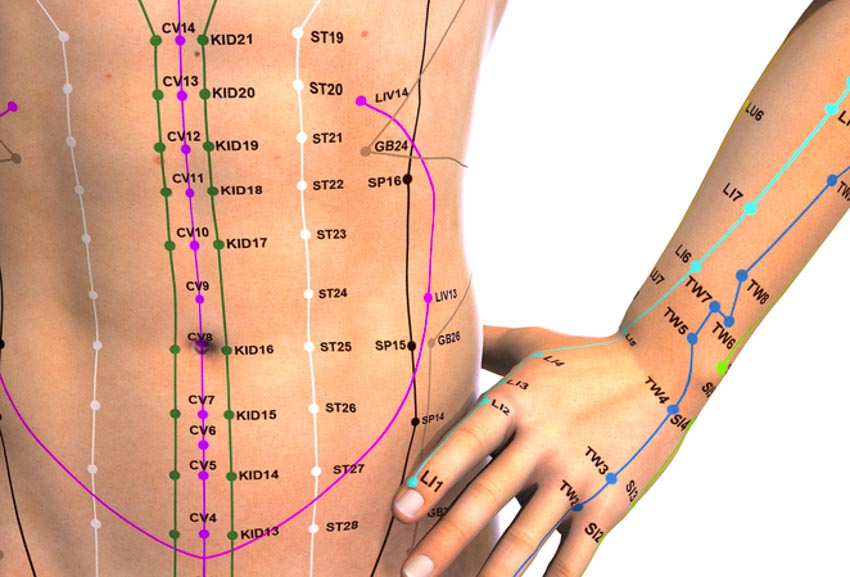This computer-generated image features a nude, gender-neutral torso viewed from the front, with the left hand resting on the hip. The image is a detailed depiction of the abdomen, prominently displaying a network of variously colored vertical lines, including purple, green, white, and blue, running down both the torso and the forearm. These lines are marked with small dots and annotated with alphanumeric codes, such as CV 8 at the belly button, CV 14 to CV 4 extending upwards and downwards, and white lines marked with ST19, ST20, ST21, and others. The lines and annotations suggest it is a type of medical diagram. The background is predominantly white, and the overall aesthetic suggests a clinical or educational purpose, despite the absence of further explanatory text. The body and hand are computer-rendered, the hand appearing lighter than the torso, which both emphasize the anatomical focus of the image.